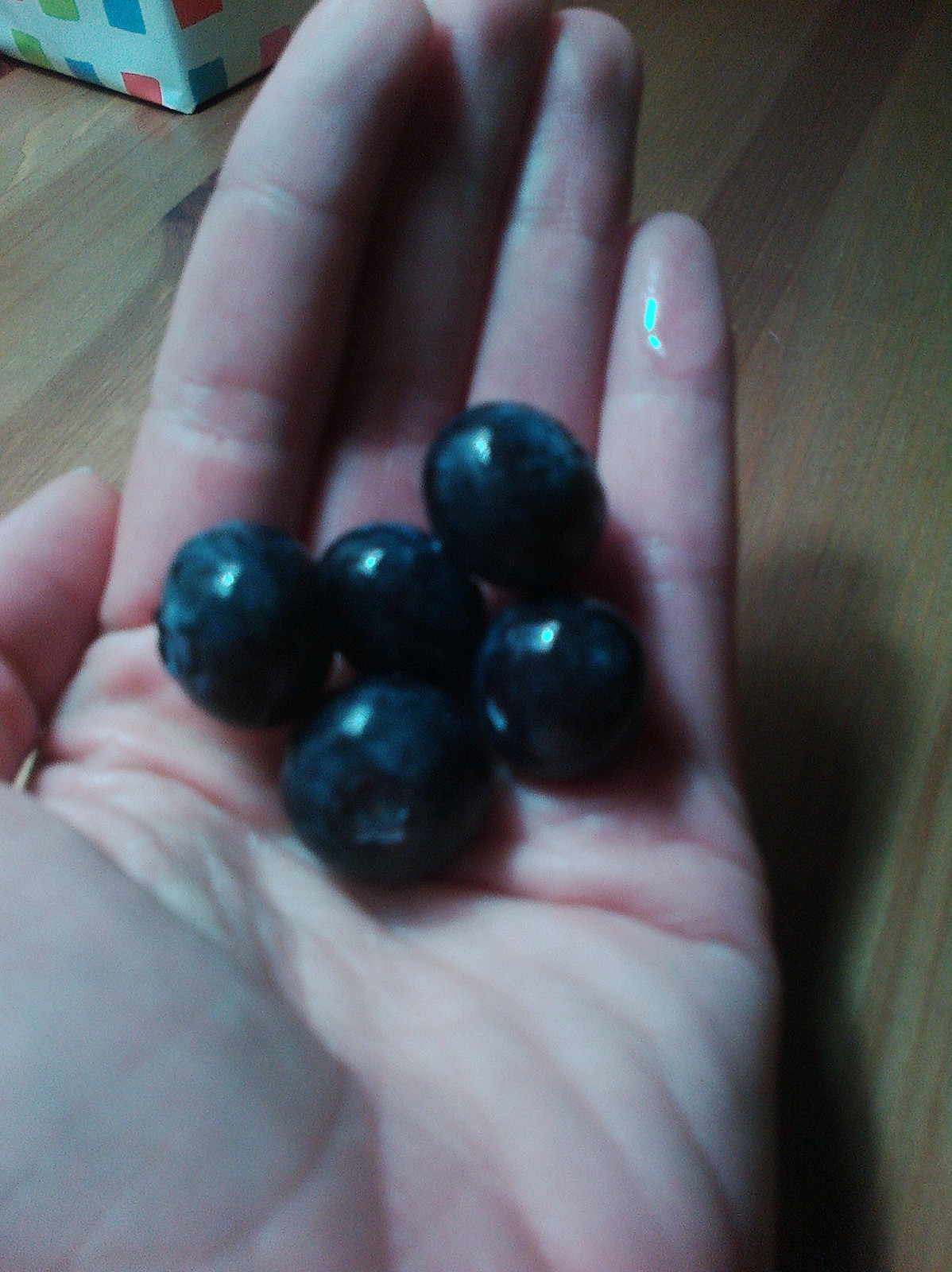The close-up image features a left hand, likely belonging to a woman, with long, slender fingers, slightly cupped to hold five almost black, plump blueberries. The index finger is slightly raised above the middle finger, casting it in complete shadow. The hand and the berries catch light from the upper left-hand corner, highlighting the glossy surface of each blueberry and creating subtle shadows on the table. There's a thick, viscous fluid, possibly a gel, on the little finger, reflecting the light. The background showcases the grain of a natural wooden table, adding a warm, rustic feel to the composition. Additionally, a highlighted box-like object can be seen in the upper left-hand corner of the image.